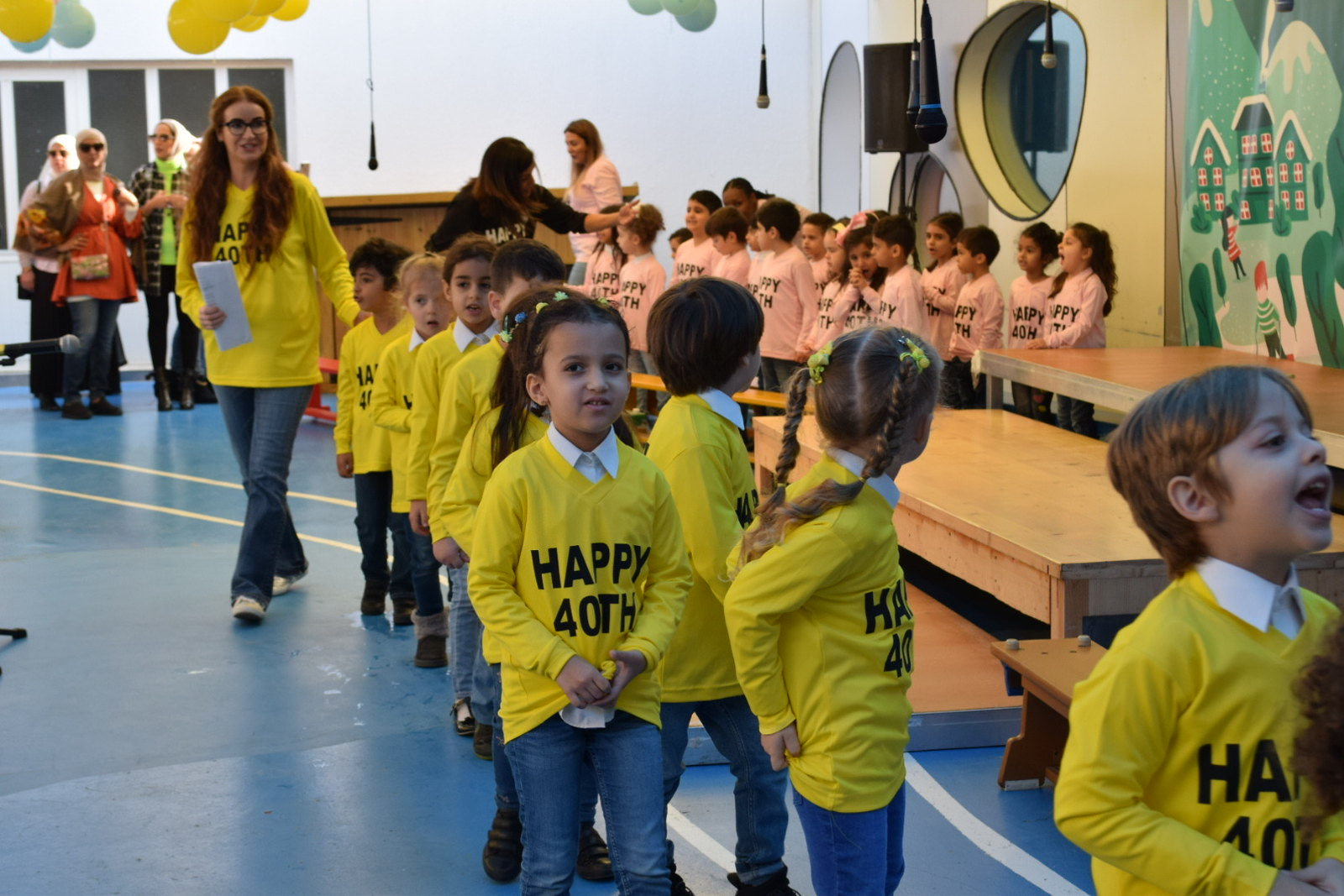This vibrant, full-color indoor photograph captures a lively school event that appears to be a children's concert in preparation. The large open room is filled with two groups of children, each consisting of about a dozen or slightly more students. One group is dressed in yellow shirts that have "Happy 40th" printed in black lettering, complemented by white collared shirts underneath and jeans. Leading this group is a woman, presumably a teacher, dressed in the same yellow shirt, directing the children who are lined up in the center of the image.

In the background, another class of children wearing pink shirts also bearing the "Happy 40th" message can be seen. An additional teacher in this group is distinguished by her black shirt featuring the same celebratory phrase. Both groups are being observed by several adults scattered throughout the room.

Suspended from the ceiling are microphones, suggesting that a children's concert or performance is imminent. The stage area on the right, adorned with wooden steps and a festive Christmas-themed banner, is currently unoccupied. Adding to the celebratory ambiance, yellow and white balloons are festively strung from the ceiling. This detailed scene captures the bustling, anticipatory energy of a school event celebrating a notable 40th anniversary milestone.